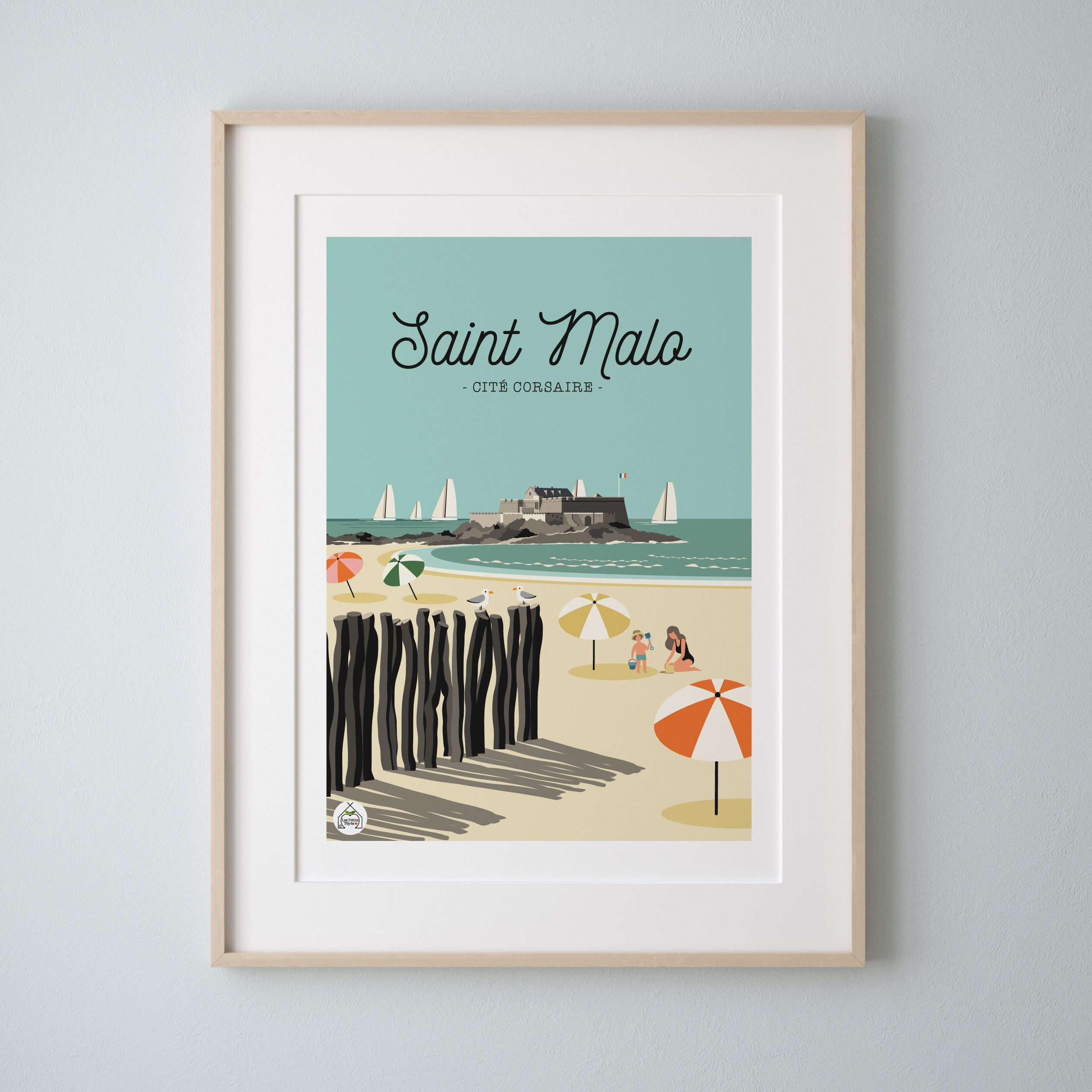This is a detailed color photograph of a framed poster print illustration hanging on a white wall. The frame is crafted from very light blonde wood and features a white mat that surrounds the image. The poster, with a light bluish-gray background, prominently displays the text "Saint Malo, Cité Corsaire." The illustration captures a lively beach scene with various elements. There are four colorful beach umbrellas in orange and white, yellow and white, green and white, and pink and orange, casting shadows on the sand. Two seagulls perch on upright wooden posts, adding a touch of coastal wildlife to the scene. In the foreground, a woman kneels beside a standing child who holds a small pail and shovel. The background showcases five sailboats gliding on the water and a rocky promontory extending into the sea, atop which sits a gray building. The overall atmosphere suggests a bright and sunny day by the beach, encapsulated within the stylish frame and mat setup.